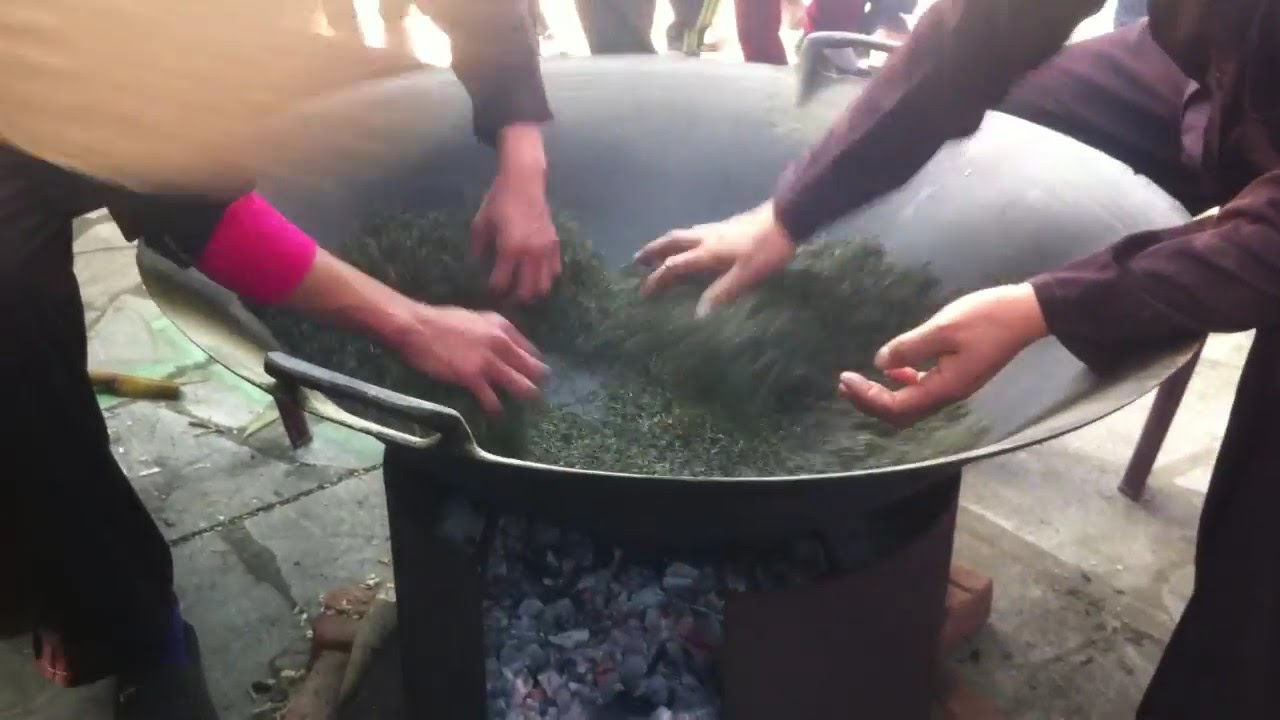In this outdoor scene, a large wok is positioned atop a coal-burning stove, with the coals glowing both white and red from the heat. The wok contains green, leafy ingredients that resemble grass. Four hands are visible, two from the left and two from the right, each belonging to different people who are actively engaged in cooking. The person on the left is wearing a maroon long-sleeve shirt and matching pants, while the person on the right has black sleeves and legs clad in black pants. Although we can't see their faces, the image captures the collaboration and focus in their culinary task. Surrounding the central action, additional legs suggest the presence of onlookers or other participants, but no further details are visible.